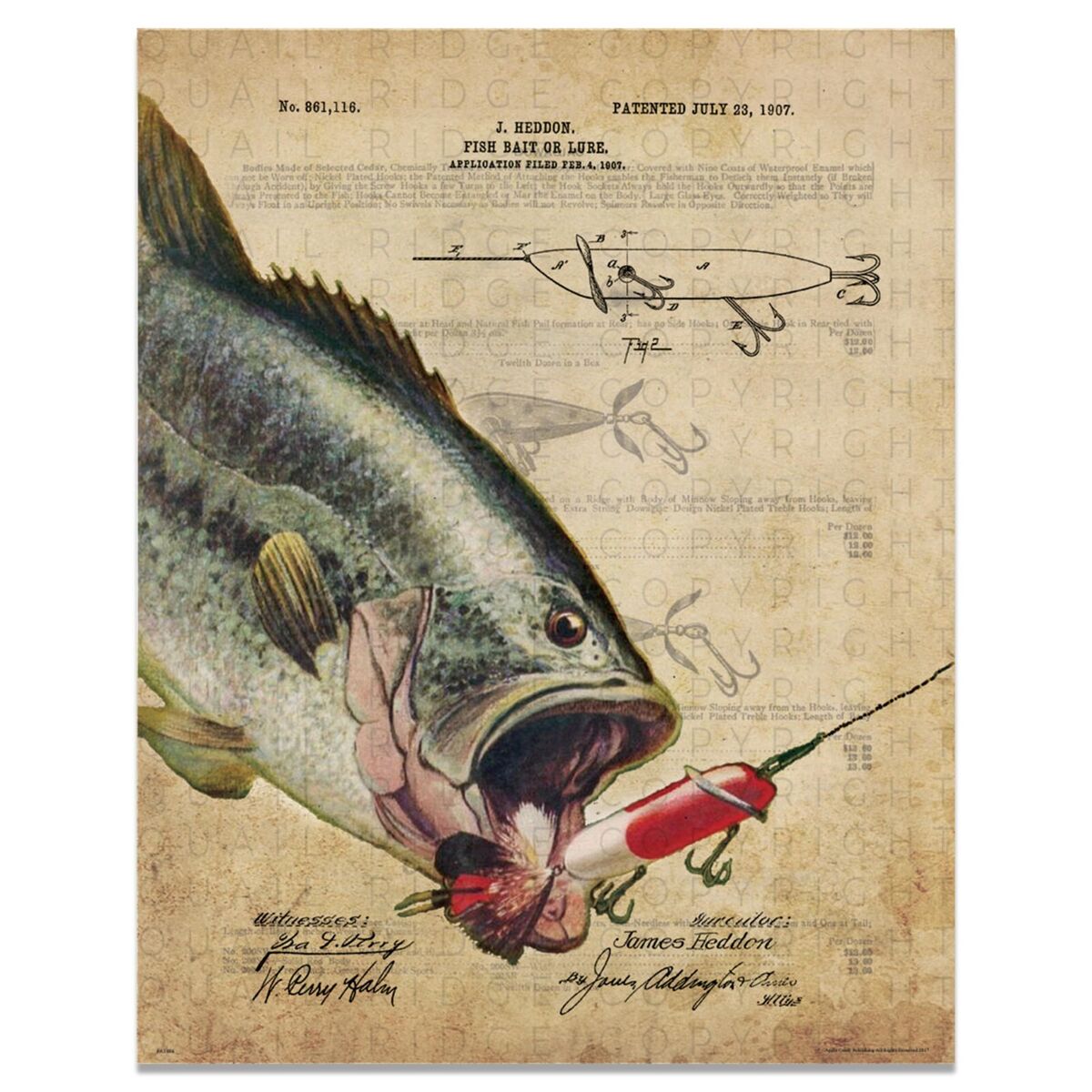This image showcases a historic patent document, dated July 23, 1907, for a fish bait or lure designed by J. Hedden, with the application initially filed on February 4, 1907. The vertically rectangular page, with a beige and brown aged appearance, features black text at the top indicating the patent number 861116. A watermark reading "Quail Ridge Copyright" is seen throughout the document. In the center, detailed illustrations include a black ink diagram of the lure and a prominent color painting. This painting depicts a large fish with a greenish-blue back and a white underbelly, its mouth wide open as it bites onto the red and white feathered lure, which is connected to a black line extending off the page. The bottom of the page contains several black signatures, possibly belonging to the inventor and witnesses.